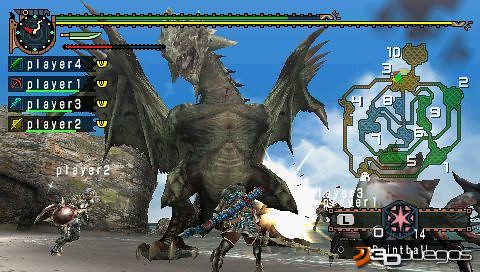The image is a screen grab from a video game featuring a climactic battle scene. Dominating the center of the scene is a large, menacing dragon with dark green and grayish scales. The dragon is being confronted by four avatars, identified as Player 1, Player 2, Player 3, and Player 4 on the left side of the screen, where their health meters are displayed. 

At the bottom of the image, three of these avatars—decked out as warriors with armor and weapons—are clearly visible. One warrior wields a weapon capable of shooting missiles, while another bears a distinctive shield adorned with horn-like projections. The warriors stand on a sandy beach where the sand meets the water, with a large rock formation on the left. In the background, the sky is a bright blue punctuated by fluffy white clouds, enhancing the dramatic and epic nature of the scene. On the right side of the screen, a map provides additional context for the in-game location. The colors in the image are vibrant, including hues of green, red, blue, and yellow, with the dragon reflecting these tones in its scales and the game interface showing green and yellow bars at the top. The text at the bottom appears to spell out "3D" and something resembling "VEGAS," adding to the game's thematic elements.